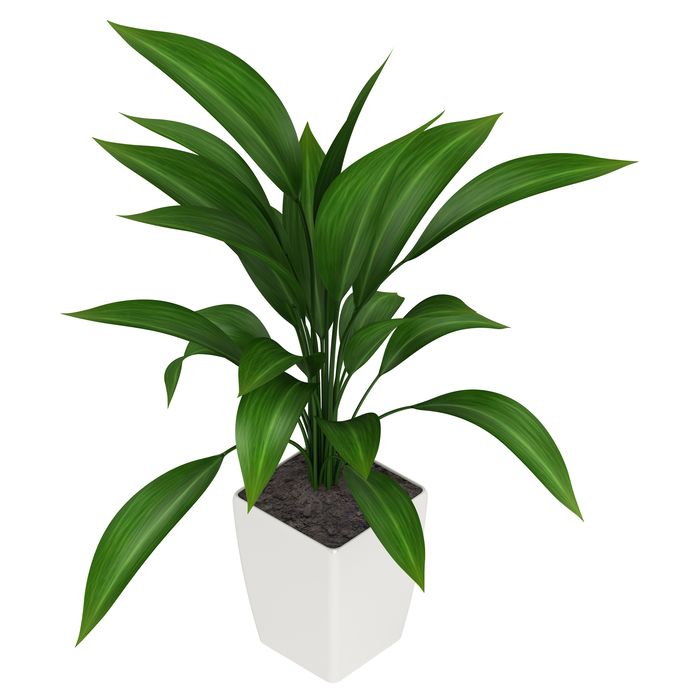The image portrays a modern, minimalist aesthetic with a prominent focus on a potted houseplant resembling a Dracaena, known for its elongated, lanciate dark green leaves. The plant, standing at approximately 1.5 feet tall, is nestled in a plain, white square pot that accentuates its vibrant foliage. The pot contains dark brown to black soil, which appears slightly clumpy and possibly artificial. The background is stark white, further emphasizing the plant's healthy and lush appearance. Despite its simplistic design, the plant's numerous leaves, some sprawling and others reaching upwards, contribute to its dynamic and naturalistic yet potentially fabricated look.